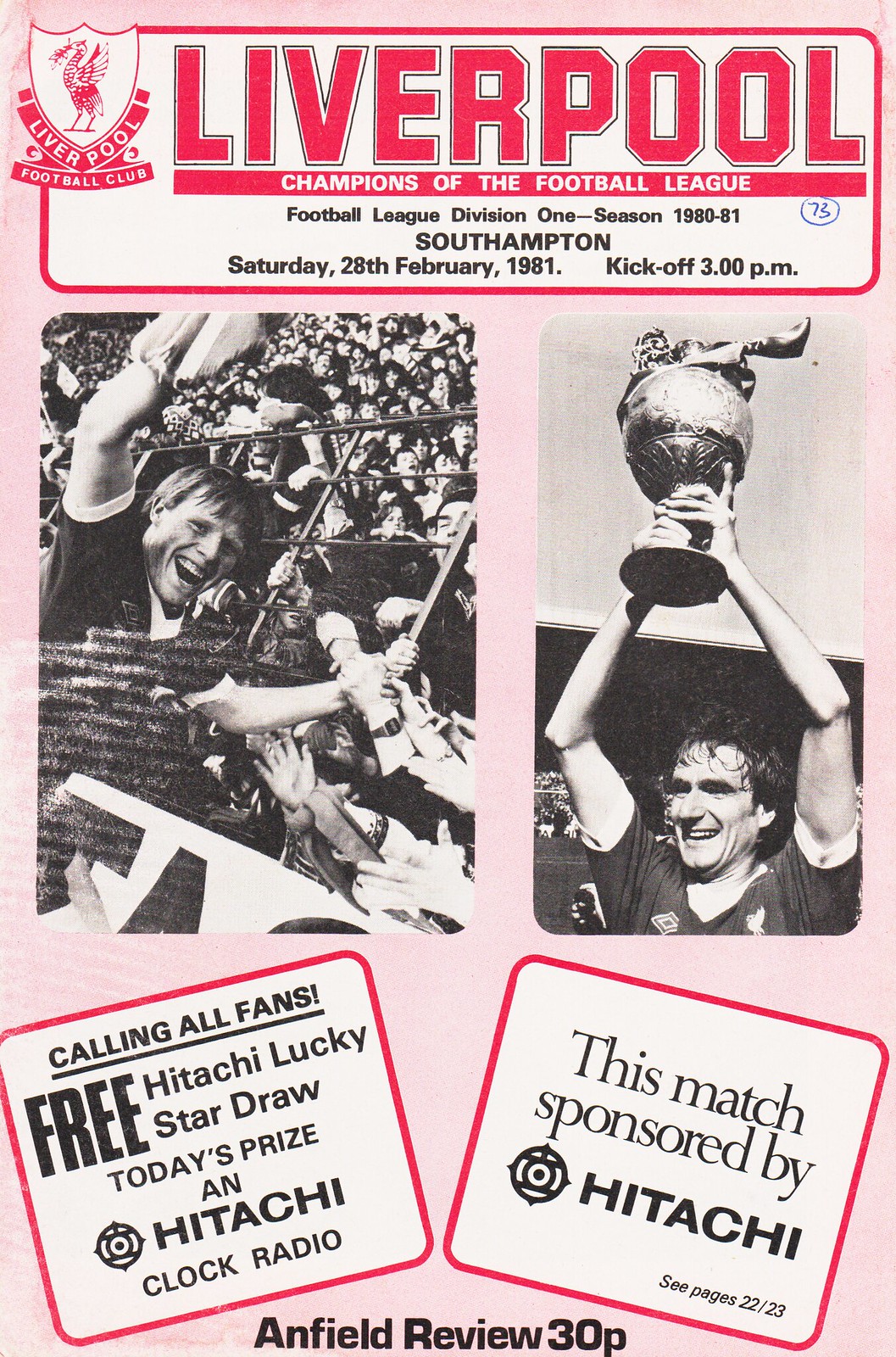This is a detailed photograph of a Liverpool Football Club pamphlet celebrating their championship in the Football League. At the top, framed in red with the distinctive red Liverpool FC logo on the left, it boldly reads "Liverpool Champions of the Football League." Directly beneath this, in smaller text, it details, "Football League Division One, Season 1980-81, Southampton, Saturday 28th February 1981, Kick-off 3 p.m."

The middle section of the pamphlet features two black-and-white photographs. On the right, a man triumphantly raises a trophy above his head with both hands, while on the left, another man is seen engaging with the fans, reaching out to grab their hands near the stands.

Below these images, the pamphlet features two red-framed boxes with additional information. The right box indicates, "This match sponsored by Hitachi, see pages 22-23." The left box announces, "Calling all fans, Free Hitachi Lucky Star draw, today's prize: a Hitachi clock radio."

At the bottom of the pamphlet, it reads "Anfield Review," all set against a pink background connected by white areas within the red squares. The overall design is clean and colorful, prominently featuring Liverpool FC’s iconic branding elements.